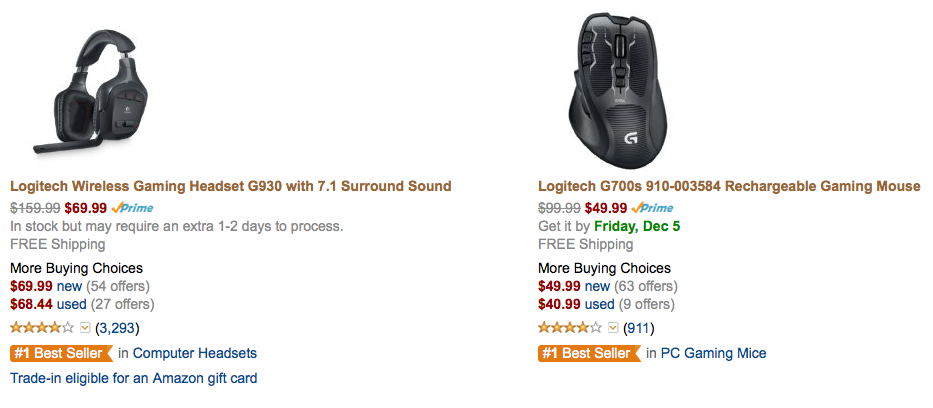**Detailed Caption:**

The image features two high-quality gaming peripherals from Logitech, currently available for purchase on Amazon.

1. **Logitech Wireless Gaming Headset G930**: This headset, equipped with 7.1 surround sound, offers an immersive audio experience for gamers. Originally priced at $159.99, it is now on sale for $69.99. Although in stock, the item may require an additional one to two days for processing, with free shipping included. The headset is highly popular, holding a four-star rating and recognized as the number one bestseller in computer headsets. Buyers can explore 54 new offers starting at $69.99 and 27 used offers starting at $68.44. Additionally, this product is trade-in eligible for an Amazon gift card.

2. **Logitech G700S-91003584 Rechargeable Gaming Mouse**: This advanced gaming mouse, initially priced at $99.99, is currently available for $49.99, with a guaranteed delivery by Friday, December 5th, and free shipping. The mouse, also a top seller in its category, is the number one seller in PC gaming mice. There are multiple purchasing options, with 63 new units priced at $49.99 and 9 used units available starting at $40.99.

These essential gaming accessories offer excellent deals and top-rated performance for gamers looking to enhance their setup.